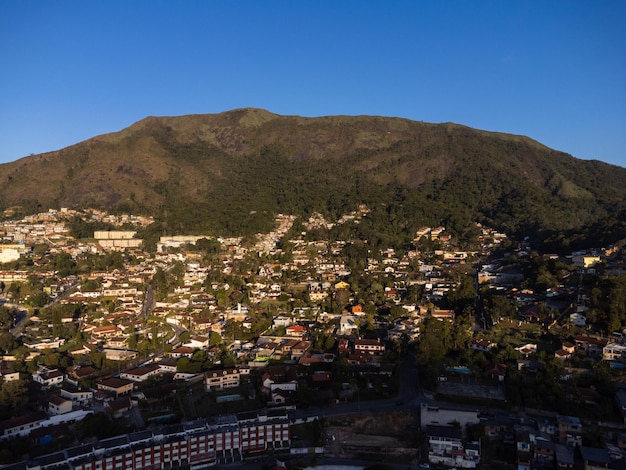This vibrant, full-color photograph captures an outdoor scene bathed in natural light on a sunny day with a bright, cloudless blue sky. The image, presented in a square format with no borders, portrays a sprawling landscape featuring a verdant mountain or large hill, devoid of snow and ice. This hillside is densely populated with dozens of homes nestled among lush, green trees, creating a picturesque community. The bottom third of the image is shaded, suggesting the picture was taken either early in the morning or late in the afternoon. In the lower-left corner, there is an indistinct structure with numerous white squares. A network of roads weaves throughout this hillside neighborhood, seamlessly integrating the settled area with the natural terrain. The overall clarity of the image is exceptional, showcasing the landscape's details and the vibrant blue sky above.